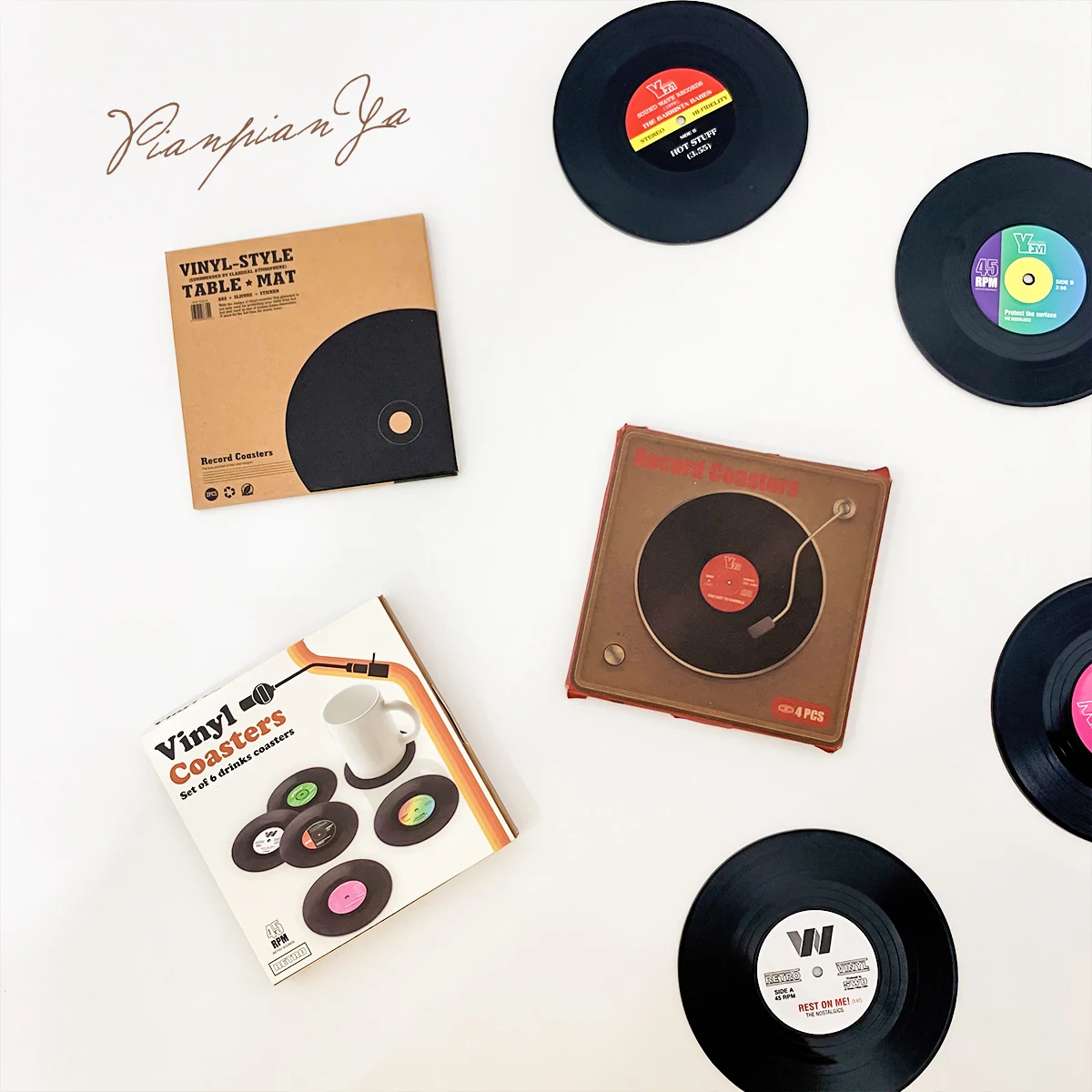The image displays a cleverly arranged advertisement featuring vinyl-themed products, which initially appear to be real vinyl records and a turntable but are actually decor items. At the center of the image is a vinyl-style table mat designed to look like a square record player with realistic detailing. Surrounding the mat are four vinyl coasters, meticulously designed to resemble authentic vinyl records, each with unique label colors. On the left side, there are two packages. The first package, labeled "vinyl style table mat," aligns with the centerpiece item. The second package, labeled "vinyl coasters," shows an image of a white mug resting on one of the coaster records. Completing the scene in the upper left corner is stylized cursive text, which appears to spell out "pian pian ja" in a golden-brown hue, adding an elegant touch to the overall presentation. All the elements are arranged in a circular pattern around the central mat, enhancing the visual appeal and coherence of the advertisement.